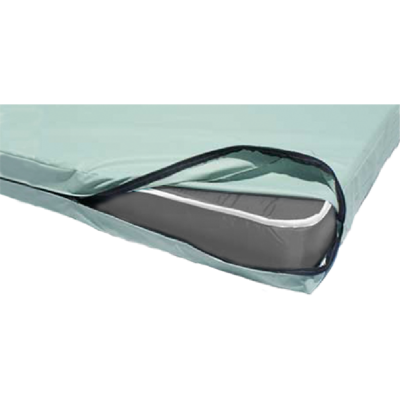The image depicts a thin, gray mattress with white edges, encased in a light green cover. The cover features a black zipper that is partially open at one corner, revealing the gray and white mattress inside. The scene is set against a plain white background, highlighting the mattress and its cover without any additional elements. The green cover with the black zipper runs along the edges of the mattress, lending it a durable and neatly enclosed appearance, while the open corner offers a glimpse of the mattress within.